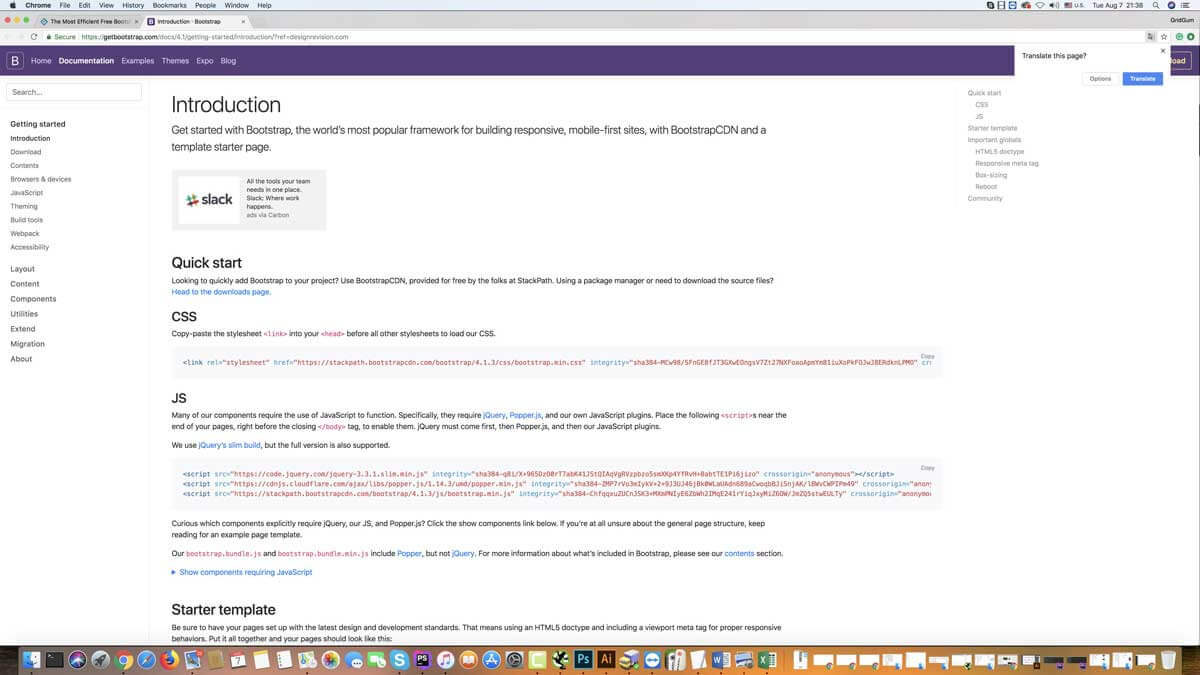In the image, we have a screenshot of a computer screen displaying the Google Chrome browser on an Apple laptop. The Chrome browser has two open tabs, and the screen is filled with a dense amount of text. In the foreground, there's a visible circular icon with white text that includes a capital "B" and words such as "Home," "Documentation," "Examples," "T," "Expo," and "On." The browser window shows a search bar and text mentioning "getting started," although much of the text is too small to read clearly. The background image appears to feature an old laptop or a planet, adding to the scene's complexity. One visible section describes the platform as "the world's most popular framework for coding," and mentions "CBM." There's black text with clickable elements leading to more content, possibly CSS-related instructions or information, emphasizing the importance of ensuring security.